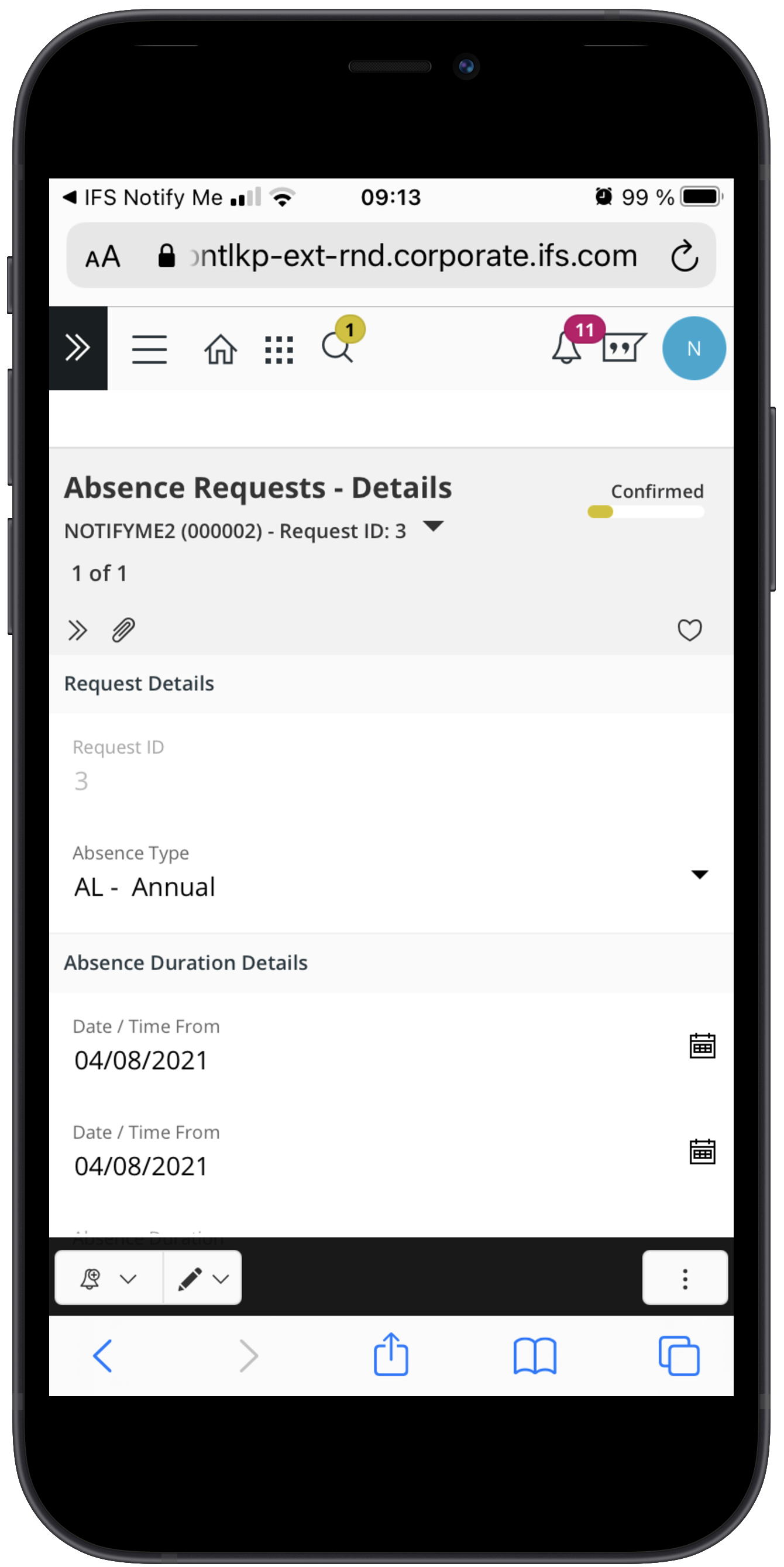A screenshot taken from a cell phone displays an app or web page with the heading "IFS Notify Me" in a white bar at the top. The status indicators show the time as 9:13 and the battery at 99%. Below the header, there is a magnifying glass icon with a notification badge indicating one alert. The main content area shows an "Absence Request Details" section with the option "Notify Me."

The details are as follows:
- Request ID: 3
- Absence Type: AL (Annual Leave)

The absence duration is specified with the same start and end date: 
- Date/Time From: 04/08/2021
- Date/Time To: 04/08/2021

This indicates a single-day absence request.